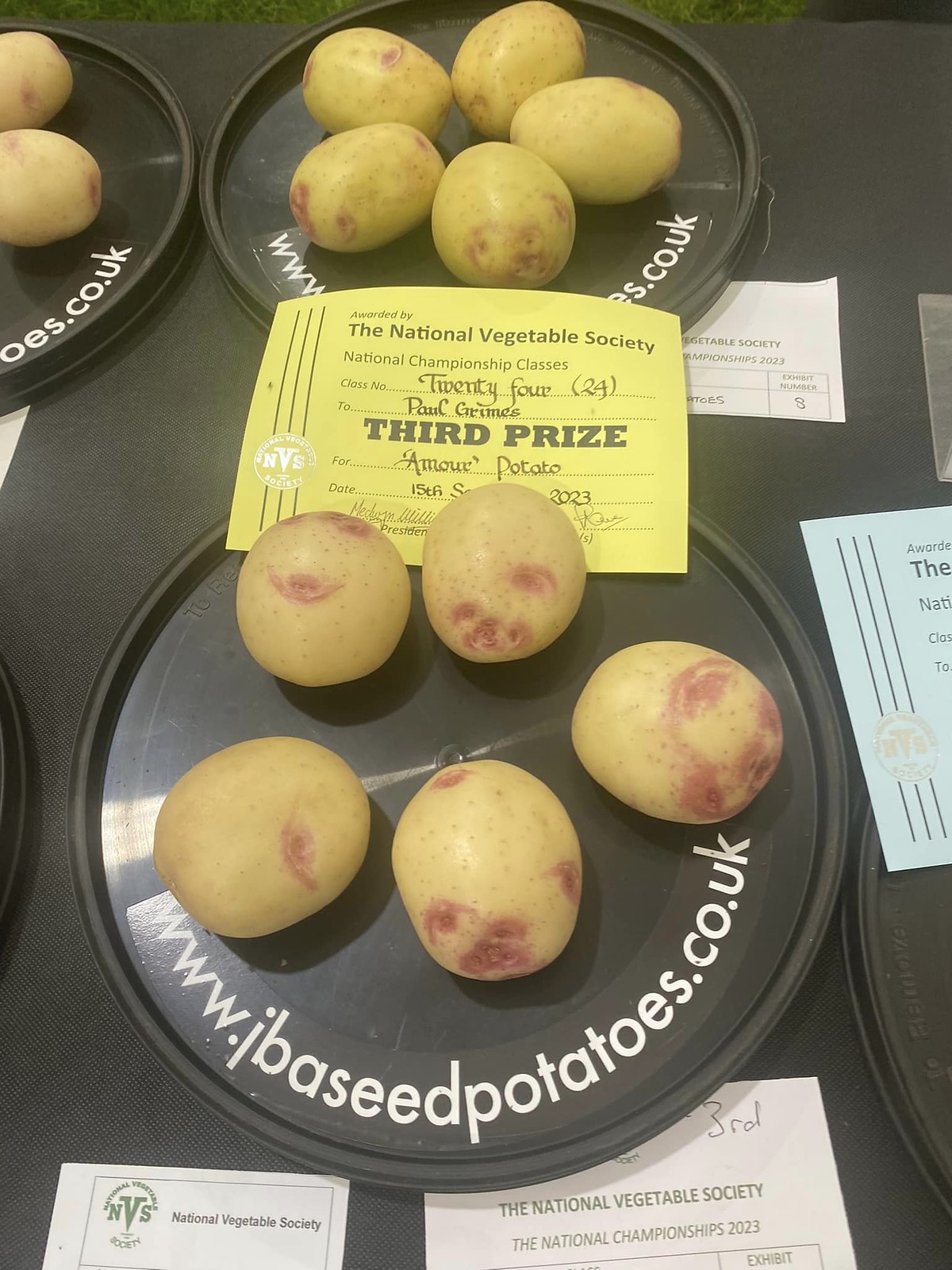In this detailed image set against a black background, we observe a scene from a vegetable growing competition. Central to the image is a black table displaying several black, circular dishes, each holding various arrangements of potatoes. One plate, placed at the center, features five tan potatoes with a partially visible text, "www...es.co.uk." Another key plate, situated at the bottom center, also displays five potatoes and bears the text "www.ibasedpotatoes.co.uk." 

Prominently placed above this bottom plate, and slightly overlapping it, is a yellow certificate that reads: "Awarded by the National Vegetable Society, National Championship Classes, Class No. 24, to Paul Grimes, Third Prize for Amore Potato." The card includes the date "15-2023," signatures, and the NVS logo.

Scattered around the plates are additional paper strips with details from the competition. The top center plate features a label mentioning the "National Vegetable Society" and "National Championship 323," alongside an "Exhibit No. 8" marker. A corresponding white strip on the third prize-winning plate bears similar accolades. In the bottom left and right sections, further documents with the "NVS" logo and mentions of the National Vegetable Society are partially visible. The array of green, brown, tan, yellow, white, and light blue colors enriches the visual composition, all amidst what appears to be an outdoor setting, suggesting a lively mid-day event.